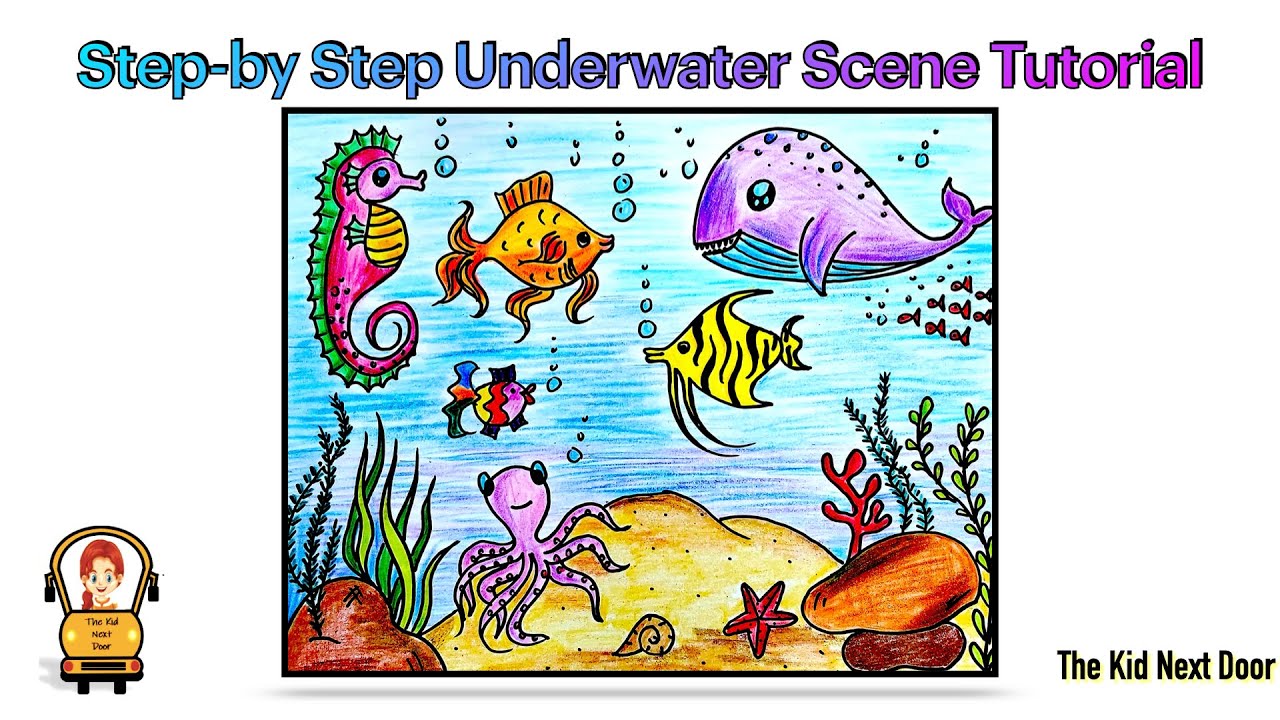The brightly colored illustration, titled "Step-by-Step Underwater Scene Tutorial," features a vibrant underwater world depicted in a cartoonish, slightly childish style. The heading at the top is presented in playful blue, purple, and pink lettering. The scene contains an array of sea creatures: a seahorse with green spines, a pink and red body, and a striped yellow stomach; a purple whale with a blue underbelly; a cheerful goldfish; an elaborate yellow angelfish with black wavy stripes; a purple and yellow round fish with zebra-like striping; and a pink octopus on the ocean floor. Additionally, the sandy ocean bottom showcases a red starfish, a brown snail, brown rocks, algae, and green plant life. All the creatures are depicted with air bubbles rising from them, adding to the underwater ambiance. On the left side of the image, there is an illustration of a little red-haired girl in a school bus labeled "The Kid Next Door." The same phrase appears again in black font with a yellow shadow on the right side of the image, creating a playful and cohesive visual composition.